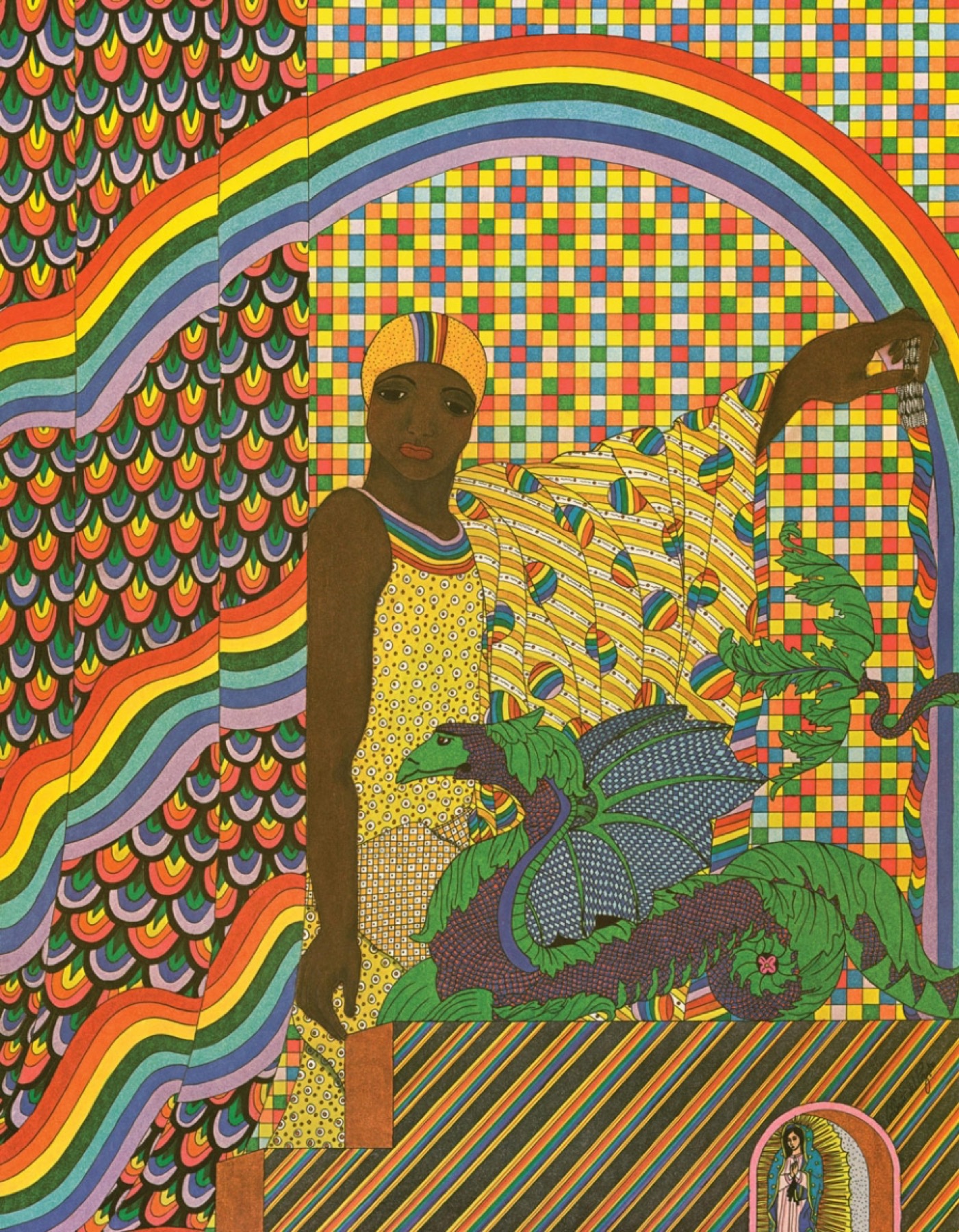The image is a vibrant and detailed illustration featuring a black woman seated within an ornate alcove. She is adorned in a yellow printed top with red and blue stripes, and her outfit includes patterns that resemble both a dress and a floral scarf. Her arm is extended, displaying fabric that echoes the colors and designs of her top. Behind her, the alcove is lavishly decorated with intricate patterns: a mosaic-tiled wall with alternating squares in shades of blue, yellow, and green; a diagonal stripe pattern below her with dark red and alternating yellow, green, and blue; and a colorful scale pattern to her left with red, yellow, orange, and dark borders. Resting in her lap is a striking blue dragon with green trim and blue and white polka-dotted wings. Adding to the mystical scene, in the lower right-hand corner, a statue of the Virgin Mary is nestled inside a cave. The background suggests a rainbow effect, starting with purple at the bottom and transitioning through the spectrum to red at the top. The woman herself is wearing a hat, completing the elaborate and colorful composition that captures a blend of cultural and fantastical elements.